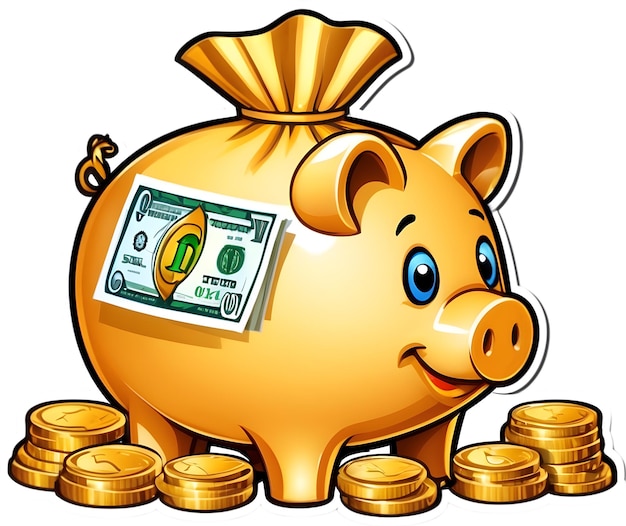This image is a detailed and stylized computer graphic of a gold-colored piggy bank with distinctive blue eyes, shaped like a traditional pig but combined with features of a money sack. The top of the piggy bank has a tied-off section with a band around it, resembling the closure of a money bag. The piggy bank is adorned with red lips, ears, a snout, and features a green and gold faux dollar bill stuck to its side, implying a playful, impressionist design rather than a realistic depiction. Surrounding the piggy bank are approximately 20 gold coins arranged in six different piles, adding to the theme of savings and wealth. The overall composition is set against a plain white background, highlighting the gold and green hues of the piggy bank and coins.